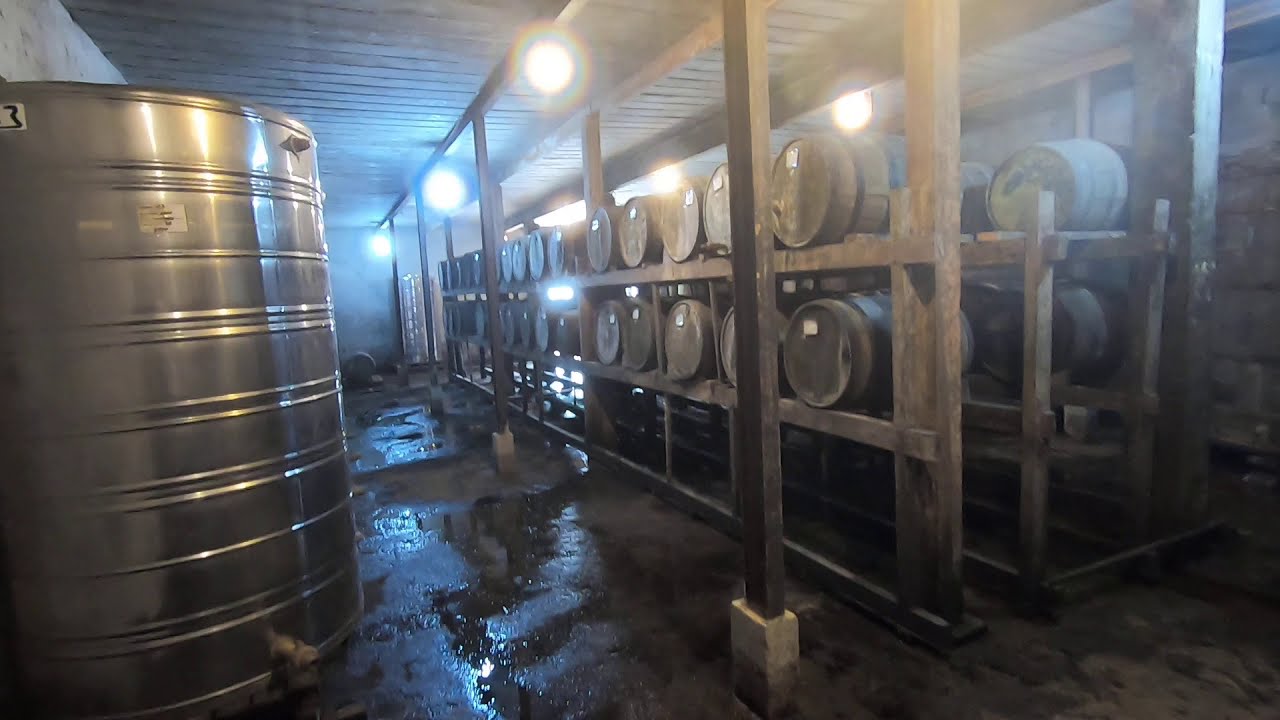The image depicts the interior of a dimly lit, damp cellar, possibly used for storing wine or beer. The concrete floor is marred with puddles, suggesting a wet environment. On the left side of the image stands a large, metallic silver barrel equipped with a spout at the bottom, conspicuously distinct from the other containers. To the right, numerous wooden barrels, roughly totaling between 20 to 30, are arranged sideways on a two-tiered wooden rack, extending into the depth of the space. The barrels appear to be labeled, although the text is illegible due to distance. The overall atmosphere is dark and dingy, with muted gray, black, and brown tones dominating the scene. However, the backdrop is punctuated by spotlights affixed to the ceiling, casting beams of light and creating a subtle rainbow effect in the image, adding a faint yet significant illumination to the area.